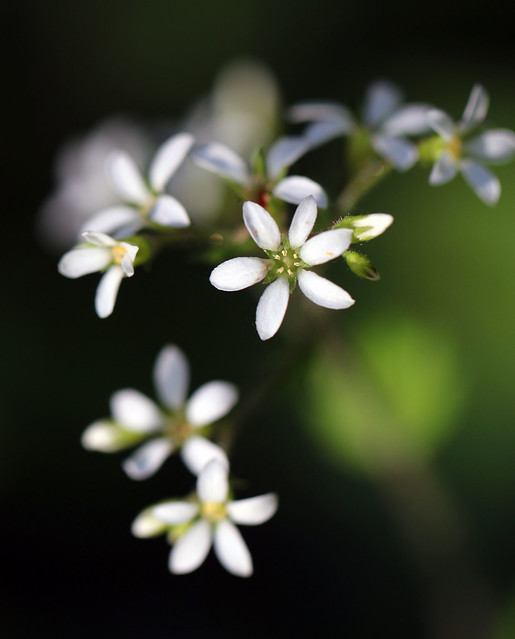This is a close-up nature photograph showcasing a cluster of white flowers against a dark, blurred background that hints at green foliage. The central focus is on one flower with six white petals surrounding a green, star-shaped center adorned with six tiny, golden-yellow pollen sacs. This flower is sharply in focus, while the surrounding flowers and unopened buds are blurred, receding into the background. The stems are mostly obscured, with a hint of green visible. Some parts of the background reveal indistinct green shapes that might be leaves, adding depth to the image. The dark, nearly black background accentuates the luminous white petals and vibrant center of the featured flower.